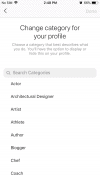An extremely blurry cellphone screenshot with large, bold black letters at the top reading "Change Category for Your Profile." The upper part of the screen contains some illegible black text, both on the left, right, and center. Below the title is an obscured paragraph followed by a gray search bar featuring a magnifying glass icon on the left. Though the text within the search bar is mostly indecipherable, it seems to pertain to configuration. Down the left-hand side of the screen is a series of eight to ten bolded black labels, although they're too blurry to read. The bottom of the image offers no additional information, rendering most of the content unreadable except for the prominent, though fuzzy, heading at the top.